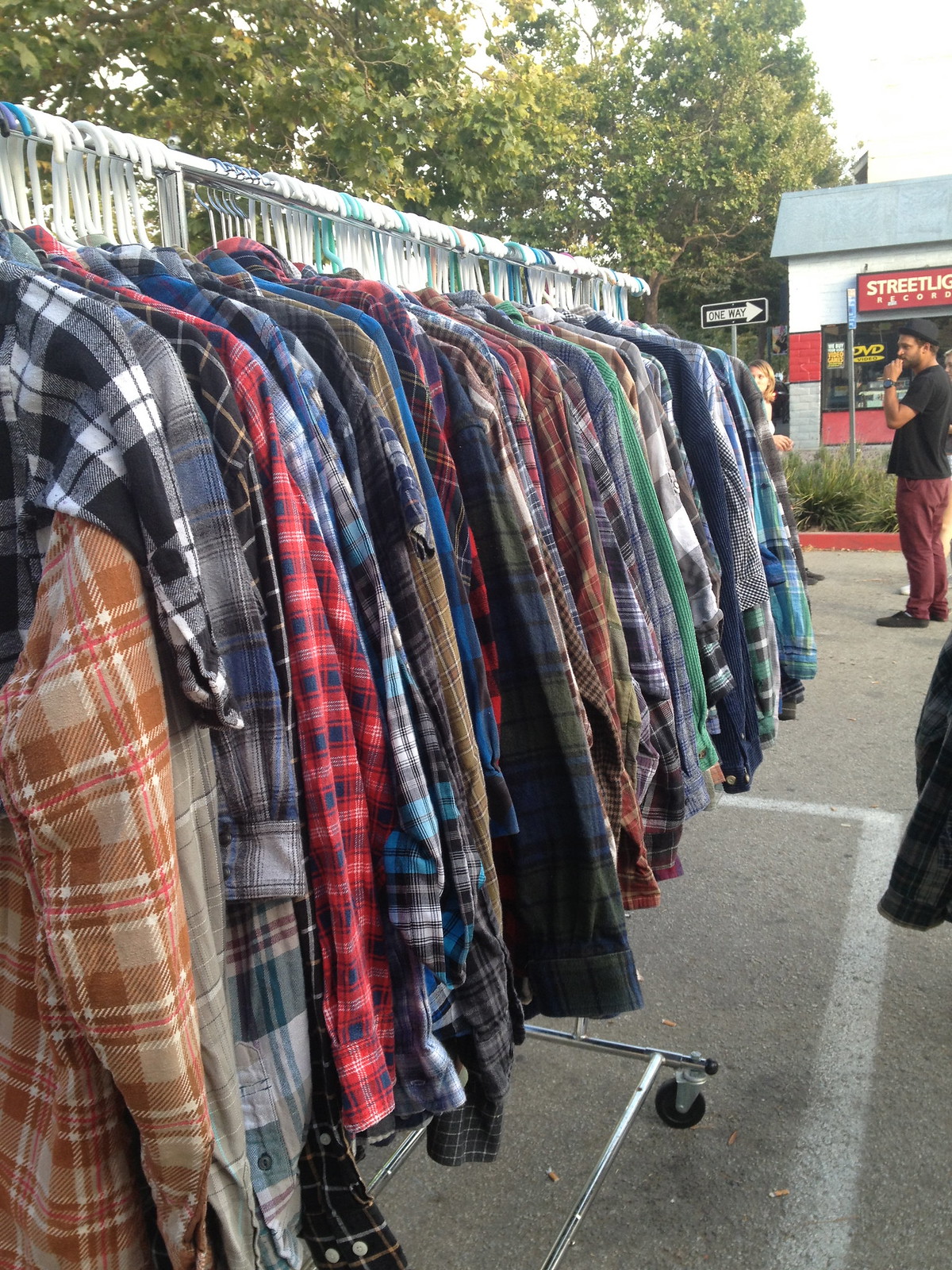This photograph captures a parking lot scene where a long, silver clothes rack is lined with various thick, long-sleeved flannel shirts. The shirts, arranged neatly on hangers, boast a range of plaid patterns and colors including camel brown, black and white, red and blue, green, and other hues. The flannel shirts are slightly thicker than standard dress shirts, providing a warmer option. In the background, two people— a man and a woman— are seen standing and conversing while observing the surroundings, enhancing the bustling street market atmosphere. The scene is set on a sunny day, and behind the rack of clothing is a store with a visible "DVD Video" logo on its window and a partially cut-off sign that may read "Streetlight Recording." Additionally, a "One Way" sign is seen along the road, with trees and a clear sky completing the backdrop.